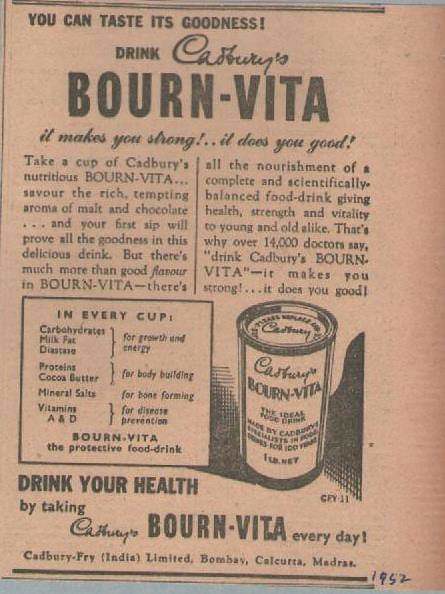The image is a vintage advertisement from 1952, reminiscent of a page from an old magazine with a brown background and black script. At the top, prominently in large font, it states: "You can taste its goodness. Drink Cadbury’s Bourne Vita." Beneath it, another tagline reads: "It makes you strong, it does you good." The ad is formatted in two columns, resembling a magazine article, and contains detailed descriptions of the product’s benefits along with an illustration of a Cadbury’s Bourne Vita container.

The descriptive text invites readers to “take a cup of Cadbury's nutritious Bourne Vita,” highlighting the rich, tempting aroma of malt and chocolate, promising that the first sip will reveal all the goodness of this delicious drink. It emphasizes that Bourne Vita offers more than good flavor; it is a scientifically balanced food drink that provides health, strength, and vitality.

A breakdown lists the nutrients in every cup: carbohydrates, milk fat for growth and energy, proteins for bodybuilding, cocoa butter, mineral salts for bone formation, and vitamins A and D for disease prevention. The advertisement also cites support from over 14,000 doctors who recommend drinking Cadbury’s Bourne Vita for its protective benefits.

The bottom of the ad notes that it was produced by Cadbury Fry, India Limited, and includes locations like Bombay, Calcutta, and Madras.